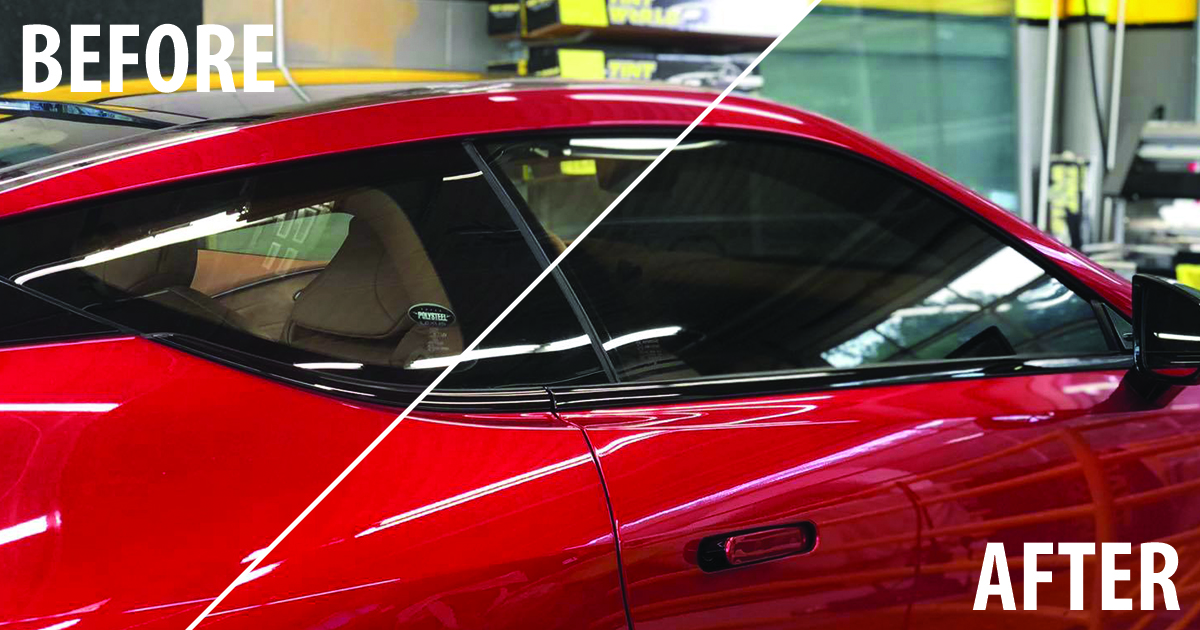This image depicts a close-up view of a bright, shiny red sports car positioned inside what appears to be an automobile shop or detailing center. The photograph is split diagonally by a white line running from the lower left to the upper right. On the top left side of the image, in all-capitalized white letters, it reads "BEFORE," showcasing the passenger side of the car, while the bottom right, also in white letters, reads "AFTER," revealing the driver’s side. Despite the intent to demonstrate a before-and-after effect of a car service—possibly detailing, waxing, or polishing—both sides of the car exhibit an equally lustrous and polished surface, making it difficult to distinguish any difference.